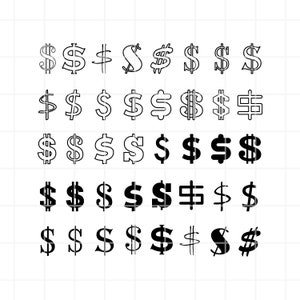The image features a collection of 40 distinct dollar signs, each rendered in various fonts and styles on a white background with faint, light gray grid lines. The designs range from thin, sleek, and elegant to bold, black, and filled-in, with some resembling pencil sketches and others taking on a whimsical or cursive appearance. A few are comprised of just black outlines, leaving the interior white, while others display unconventional, squared-off shapes that deviate from the typical curved S form. The dollar signs are organized into five columns and eight rows, reminiscent of a tattoo flash sheet or font selection guide, showcasing a diverse array of artistic interpretations of the iconic money symbol.